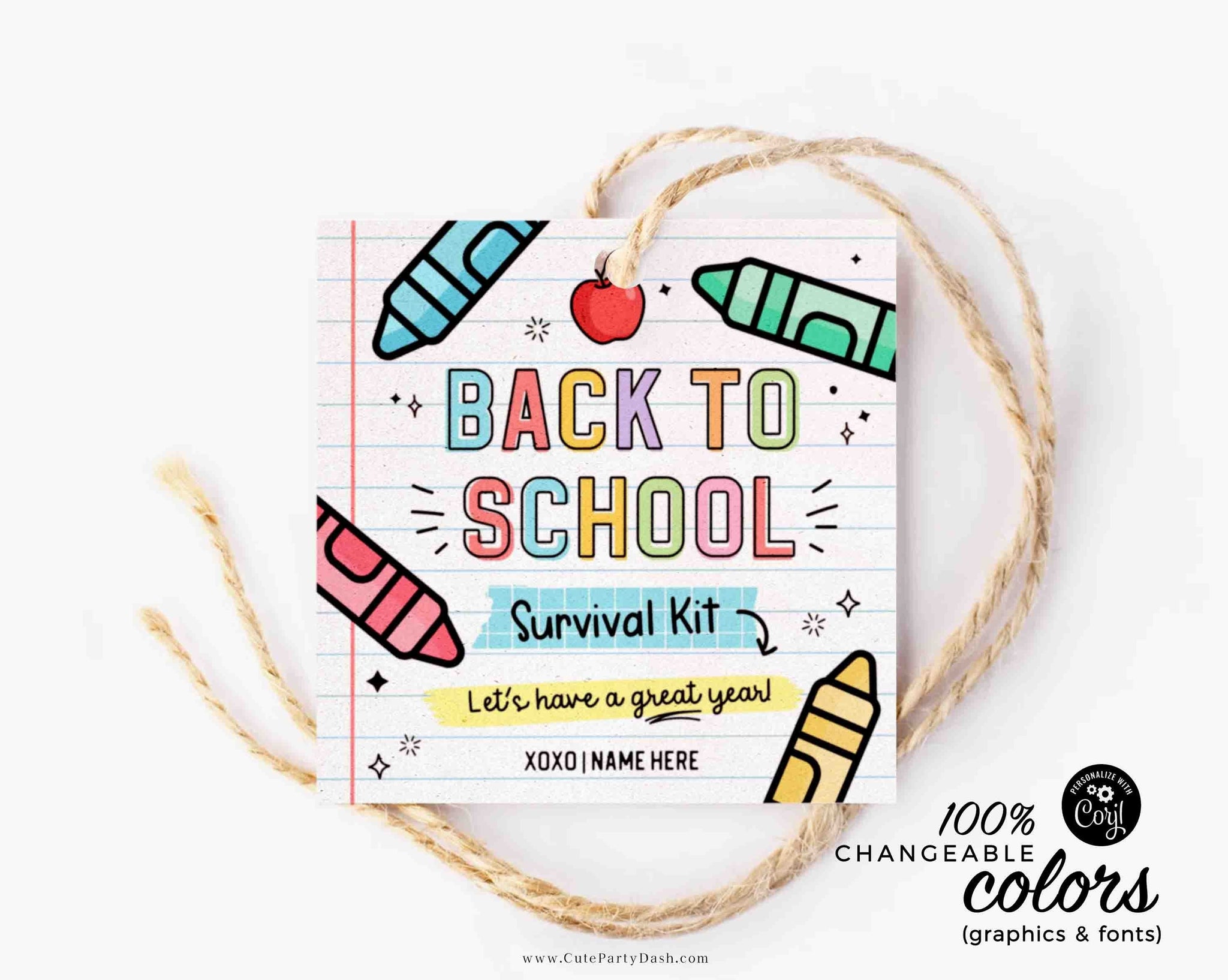The image displays a neatly centered piece of paper resembling lined notepaper, labeled "Back to School Survival Kit," accompanied by the message "Let's have a great year" and signed "XOXO name here." The paper is adorned with an apple at the top near a hole cut for a piece of twine, which loops from the top, trailing down to the bottom middle. Scattered around the paper are four crayons in blue, green, red, and yellow, pointing in various directions. A small logo is positioned at the bottom right corner. The design is colorful, featuring shades of blue, green, red, yellow, tan, black, and white. The tagline at the very bottom proclaims, "100% changeable colors, graphics, and fonts," with a website address, www.cuteparty-.com. The overall style suggests this is an advertisement for a customizable back-to-school survival kit, likely being sold online.